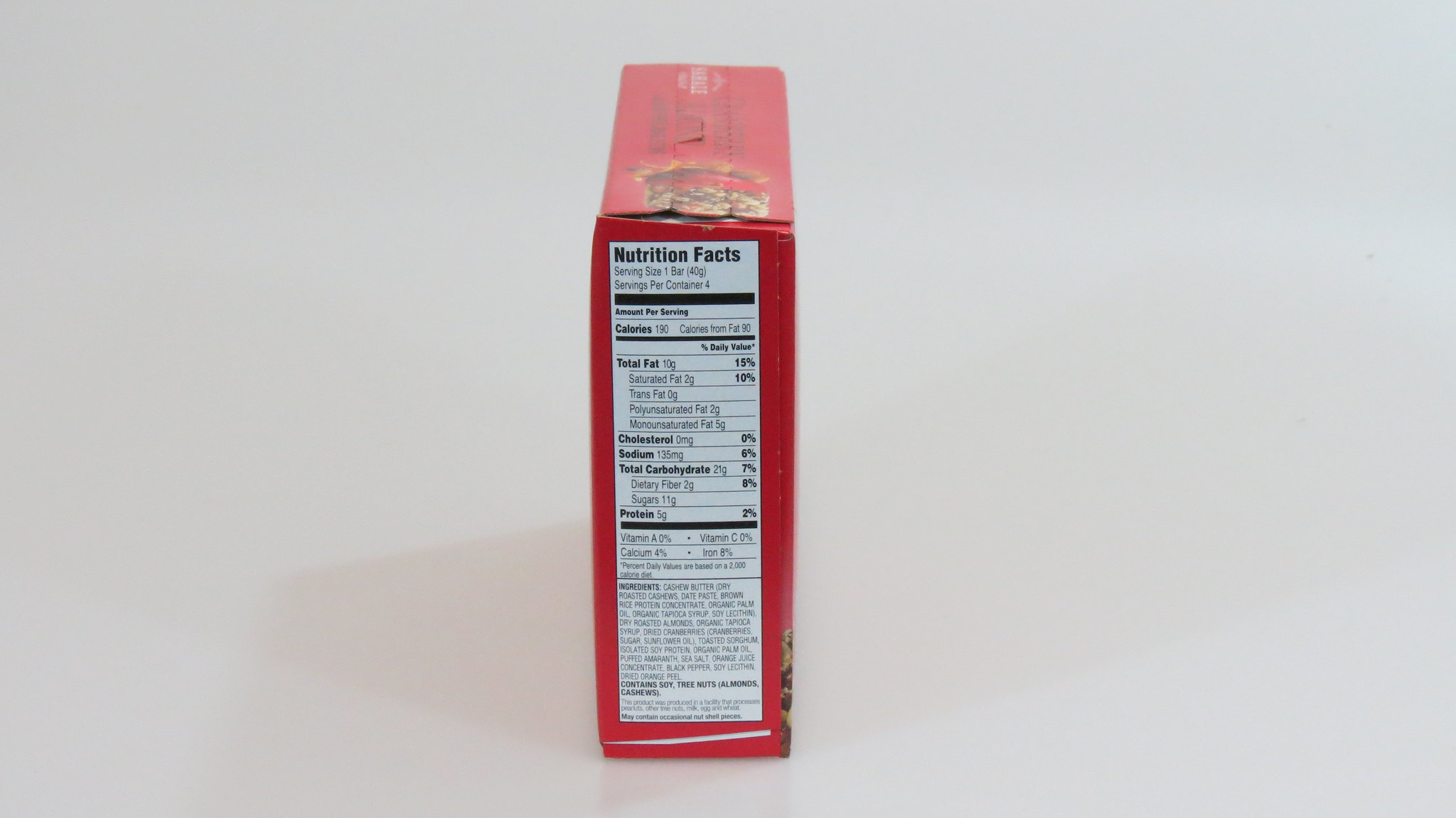This photograph showcases a small red box, similar to those found in grocery stores, set against a grayish or light bluish surface. The box's main visible feature is the nutrition facts label on its side, presented on a white background with black text. The detailed label highlights a serving size of one bar, 40 grams, with four servings per container. Key nutritional values include 190 calories, 90 of which are from fat, 10 grams of total fat (15%), 2 grams of saturated fat, 0 grams of trans fat, 2 grams of polyunsaturated fat, 5 grams of monounsaturated fat, 0 milligrams of cholesterol, 135 milligrams of sodium, 7% total carbohydrates, and 5 grams of protein. The box mentions "cashew butter" as the first ingredient, suggesting it contains some form of food product, possibly bars. The box appears unopened as indicated by an intact pull tab at the top.